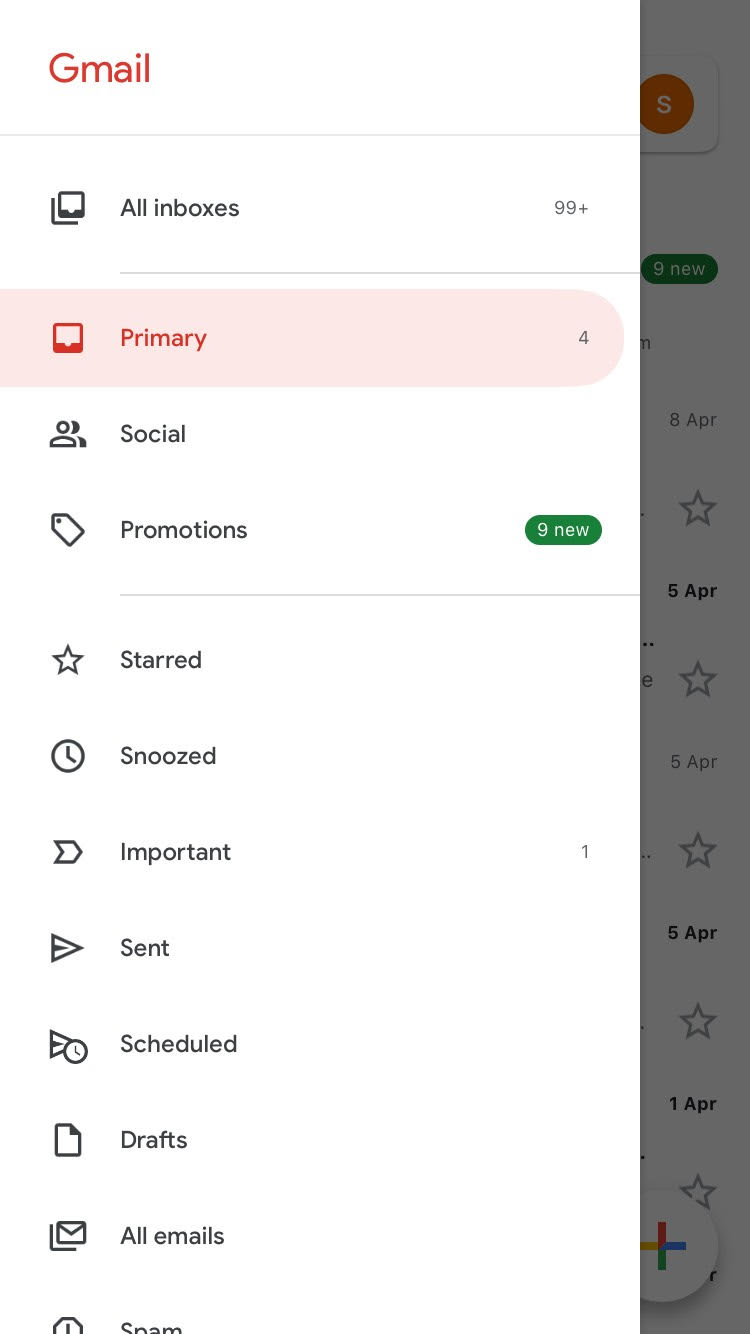This screenshot captures a detailed view of a Gmail inbox on a smartphone. The email account is currently displaying the primary sections and multiple tabs at the top. 

The primary toolbar shows a total of 99+ unread emails and a highlighted "Primary" tab with 4 unread messages. Below this, the following tabs are visible:

1. **Social** - represented by a two-person icon.
2. **Promotions** - identified by a tag icon, showing 9 new emails.
3. **Starred** - marked with a star icon.
4. **Snoozed** - indicated by a clock icon.
5. **Important** - denoted by a banner icon.
6. **Sent** - displayed with a right-facing arrow icon.
7. **Scheduled** - also displayed with a right-facing arrow clad in a clock icon.
8. **Drafts** - shown with a piece of paper icon.
9. **All Emails** - represented by an envelope icon.
10. **Spam** - marked with a stop sign icon.

The main display is currently focused on the Promotions tab, which is highlighted against a gray shade background.